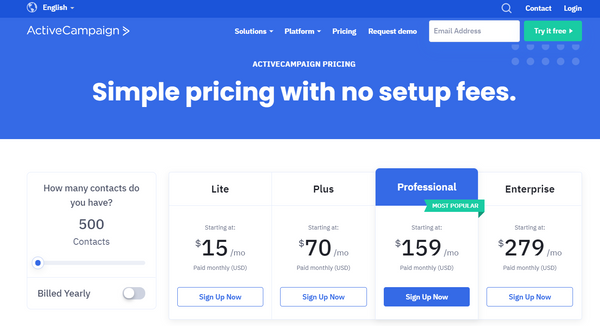This screenshot captures the pricing plans page of the ActiveCampaign website in great detail. The top-most section features a blue header displaying the ActiveCampaign logo on the left with options for language selection (English), Contact, and Login on the right. Just below this header, a navigation bar provides links to areas such as Solutions, Platform, Pricing, and Requests for Demo. Additionally, there is a search icon and an email sign-up field accompanied by a green button labeled "Try It for Free."

The main banner beneath the navigation bar has a blue background and prominently showcases bold white text that reads, "Simple Pricing with No Setup Fees." Directly below this, smaller text reiterates, "ActiveCampaign Pricing."

The core of the page is dedicated to a detailed section displaying four columns of pricing plans, tailored to different user needs. Prior to listing the specific plans, there's a feature allowing users to input and select the number of contacts they manage, affecting the pricing details.

The pricing plans are as follows:

1. **Light Plan** - Priced at $15 per month.
2. **Plus Plan** - Priced at $70 per month.
3. **Professional Plan** - The most popular option, priced at $159 per month.
4. **Enterprise Plan** - The most comprehensive offering, priced at $279 per month.

The layout maintains a clean and straightforward design focused on helping users easily understand and select their desired plan without any confusion.